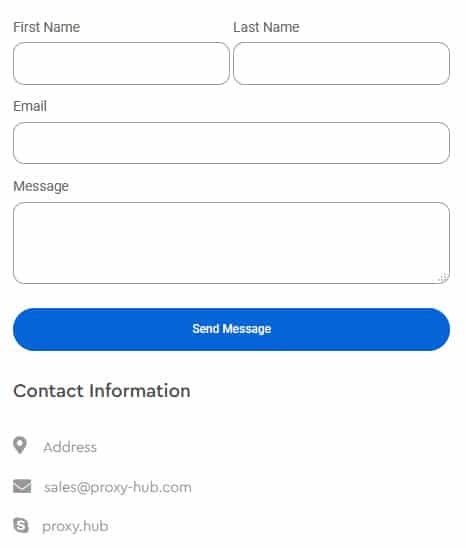This image depicts a clean, user-friendly form designed to collect personal information and messages. The background is entirely white, lending the form a minimalist and modern aesthetic. 

1. **Form Fields:**
   - The topmost section includes two fields labeled "First Name" and "Last Name" in gray letters. Each field is outlined with a thin gray line and has rounded corners, emphasizing a sleek design.
   - Directly below is a similarly styled field for "Email," spanning the full width of the form.
   - The next section contains the label "Message" followed by a larger text box for users to input their messages. This text box also features a thin gray outline with rounded corners.

2. **Submission Button:**
   - Under the message field is a prominent blue button. This button stretches across the entire width of the form and features rounded edges. In its center, the white text reads "Send Message," indicating the call to action.

3. **Contact Information:**
   - Below the submission button, the text "Contact Information" is displayed in dark letters aligned to the left.
   - The contact section includes:
       - A gray location symbol followed by the word "Address."
       - An envelope icon next to the email address "sales@proxy-hub.com."
       - A white "S" on a gray background next to the text "proxy.hub."

The overall layout is simple and intuitive, focusing on ease of use and accessibility.